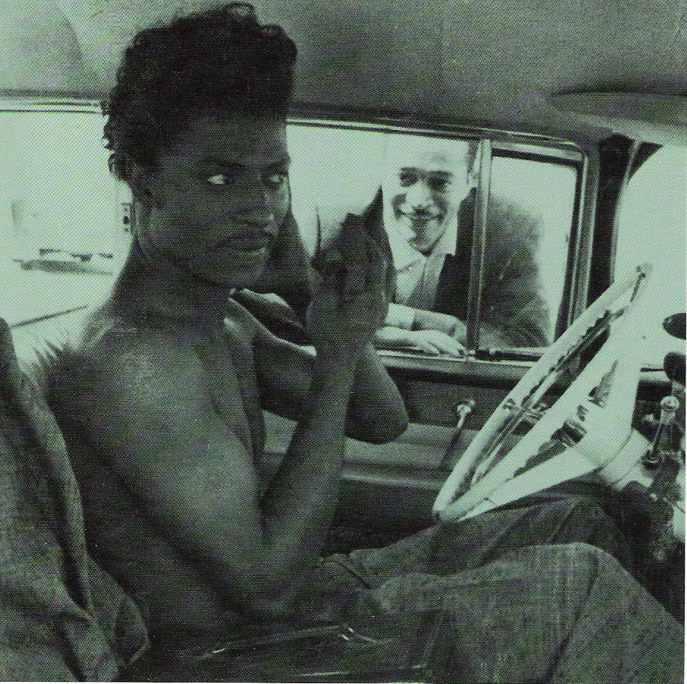A black and white photograph from the 1960s or 70s captures a candid moment between two black American men involving an old automobile. The image, with a slightly bluish-gray tinge, is taken from the perspective of the passenger seat, focusing chiefly on the shirtless driver. He has dark-toned skin, a poof of curly hair, and a thin mustache, appearing to perform some kind of grooming with the help of a mirror, possibly applying something to his face. The driver, wearing trousers, exudes a sense of ease and positivity through his smile. Leaning into the open window from outside the car, the other man, of lighter complexion, wears a suit jacket without a tie. He is smiling warmly at the driver, suggesting a friendly, cheerful interaction. The vehicle itself has an older design, emphasized by its distinctive vintage steering wheel. This nostalgic scene is rich in detail, evoking a sense of camaraderie and simple joy amidst the ordinary.